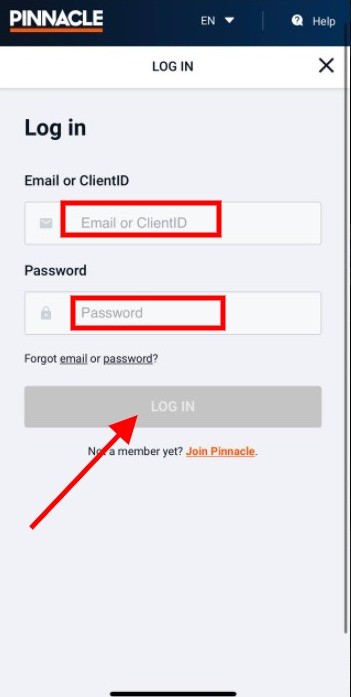This image is a color, portrait-format screenshot taken from a mobile phone, depicting the login page of an app or website branded as "PINNACLE." The brand name appears in all caps, with bold white letters "P-I-N-N-A-C-L-E" underlined by an orange line. This branding is displayed on a navy-blue banner occupying the top portion of the screen.

On the upper left of the navy-blue banner, there is an option to toggle the language settings, presently showing "EN" (for English) with a downward-pointing arrow indicating the availability of other language options. Additionally, on the top right section of the banner, there is a help button symbolized by a question mark.

The main content of the screenshot focuses on the login functionality. Two input fields are prominently shown: one for either an email or client ID, and the other for a password. Both input fields are highlighted with conspicuous red squares, seemingly to guide users on where to enter their information. Beneath these fields, there is a "Forgot email or password?" link for recovery options. Finally, a prominent login button is presented at the bottom of these input sections, which users are meant to tap after entering their credentials. No other content is visible on the page.